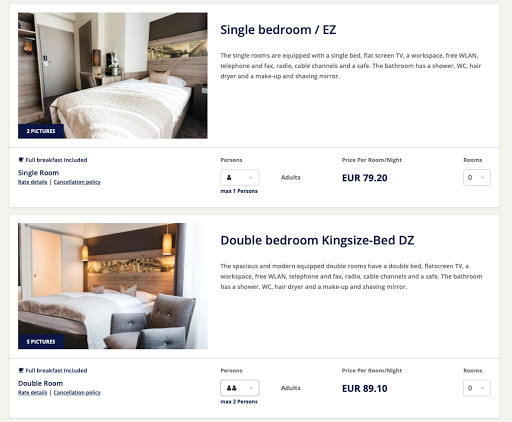This image appears to be a section of a hotel booking website presenting different room options. On the left side of the image, two photographs showcase different bedroom styles within the hotel. 

The top photograph depicts a single bedroom, furnished with a large bed adorned in white and gray sheets. Surrounding this image is a white background with black text. To the right of this top photograph, there is a description that reads: "Single Bedroom / Easy. The single rooms are equipped with a single bed, flat screen TV, workspace, and free WLAN." Beneath this description, at the bottom center of the photograph, the price is listed as €79.20.

The bottom photograph shows a double bedroom featuring a king-size bed, similarly dressed in white and gray sheets, but with a slightly varied room style compared to the single bedroom. Below this image, the text describes: "Double Bedroom, King Size Bed, DZ." Further details of the room can be found beneath this description. At the bottom center of the second photograph, the price is listed as €89.10.